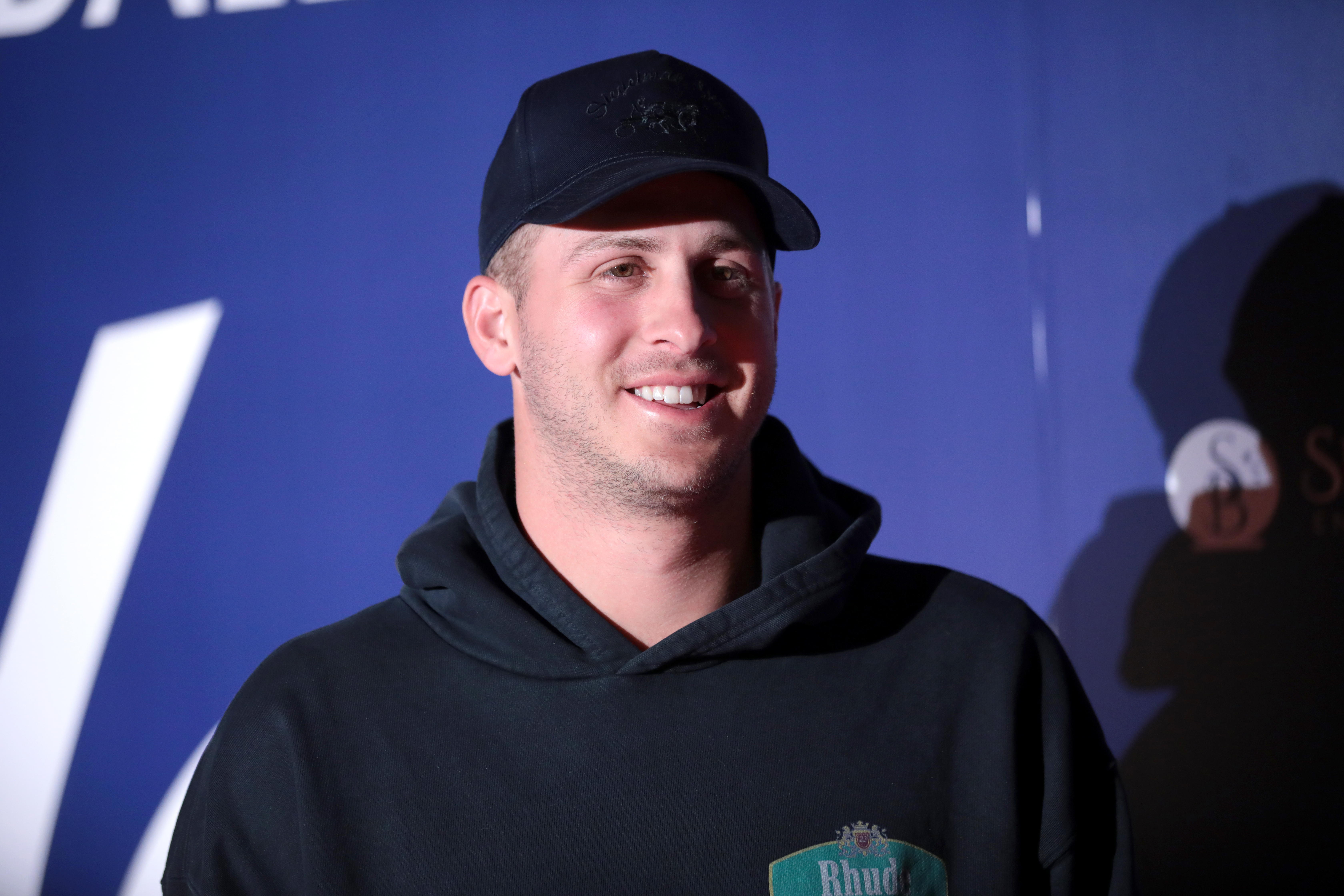The photograph showcases a man from his upper shoulders upwards, centered against a solid blue background with partially visible, cut-off logos around the edges. He is dressed in a black pullover hoodie, which features a green rectangular logo with a yellow border and white letters that read "B-H-U-D" on the left chest area. He is also wearing a black baseball cap with the brim facing forward. The man is smiling, revealing the top row of his white teeth, and his eyes are directed to the right of the image while his body faces forward. The photograph appears to be taken indoors under artificial lighting, as indicated by the slight reflections on his cheeks. The man has some stubble on his face, adding to the detailed depiction of him in this indoor setting.